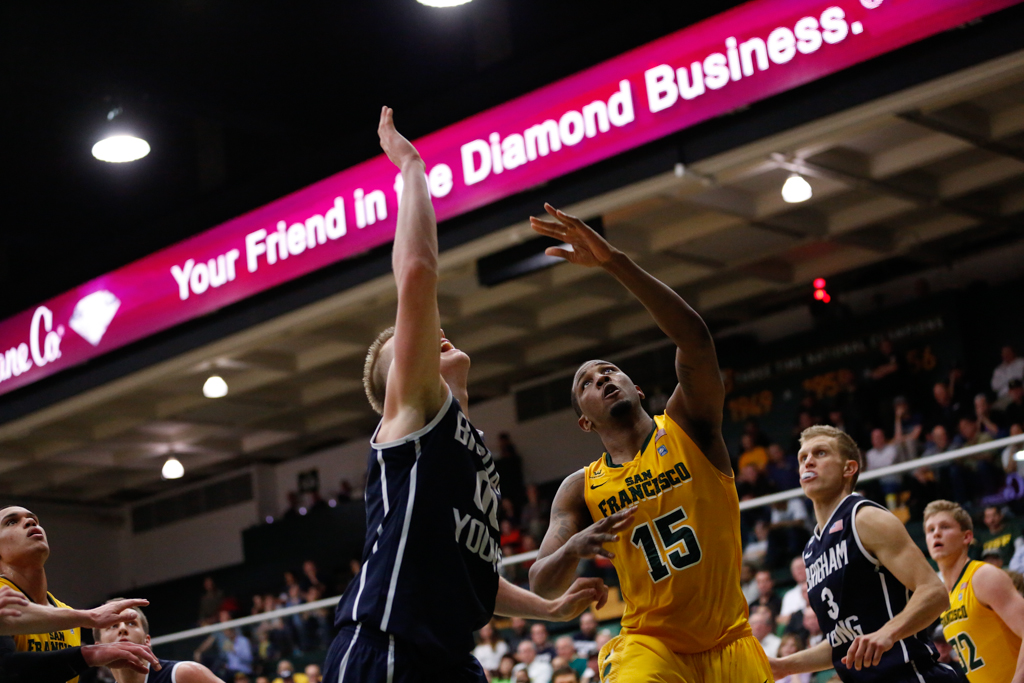The indoor photograph captures an intense moment in a basketball game, focusing on two players leaping into the air with their hands outstretched, seemingly reaching for an unseen ball above the frame. The player to the left, an African American wearing a yellow San Francisco jersey numbered 15, competes fiercely against a Caucasian player in a blue and white uniform. Surrounding them, other players can be observed: a player in yellow with the number 32, and another in blue and white with the number 3. The lower-left corner of the image features additional players, one in yellow and another in blue. Behind the action, a packed stadium full of spectators forms a blurry backdrop, emphasizing the crowd's excitement. Above the spectators, a prominent red banner reads "Your Friend in the Diamond Business," accompanied by an indistinct logo to its left, all illuminated by bright lights hanging in the dark area above.